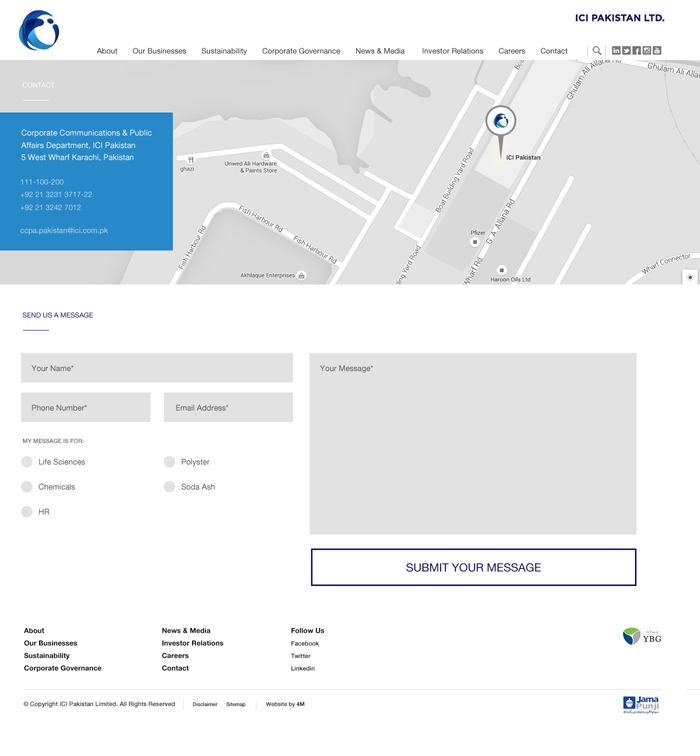"Corporate Communications and Public Affairs Department at ICI Pakistan: The map displayed in gray and white pinpointing the location of ICI Pakistan. The company's name, 'ICI Pakistan Limited,' is highlighted in blue. There is a section inviting users to 'Send us a Message,' featuring fields for 'Your Name', 'Your Phone Number', and 'Your Address,' all contained within gray boxes. Additionally, there is a larger gray box designated for 'Your Message.' Users can specify the department their message pertains to, such as Life Sciences, Chemicals, HR, Soda Ash, or Polyester. The form concludes with a blue 'Submit Your Message' button."